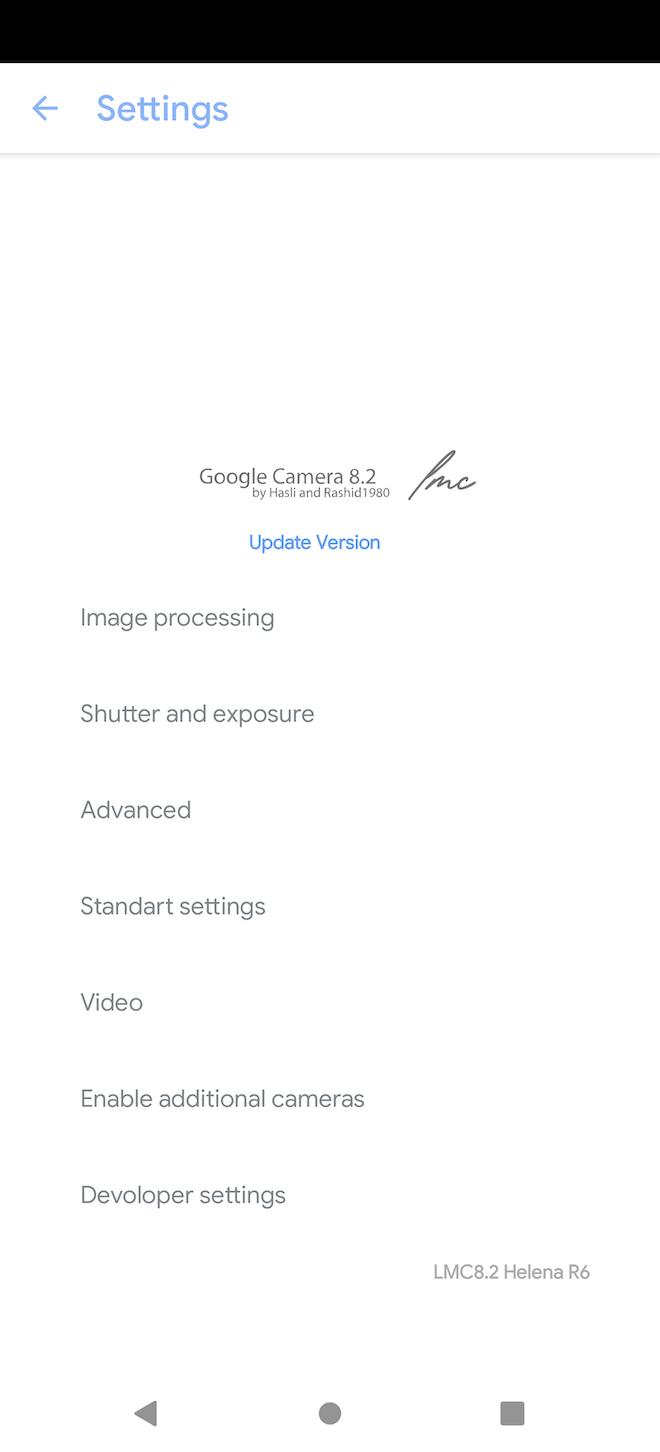Screenshot of the Google Camera settings screen, featuring a predominantly white background with a black header bar labeled "Settings." Below the header, in blue text, is the option to "Update Version," indicating "Google Camera 8.2." The screen also lists various camera settings, including "Image Processing," "Shutter Exposure," "Advanced," "Standard," "Art," and "Video," all of which are labeled as "Enabled." Additionally, there are options for "Additional Cameras" and "Developing Settings." A gray arrow icon, a gray solid circle, and a gray solid square are also visible on the screen. Towards the bottom, it reads "LMC82HelenaRX." The screenshot is devoid of any additional elements, except for a small scribble resembling a signature in the lower section, which appears to say "PMC."